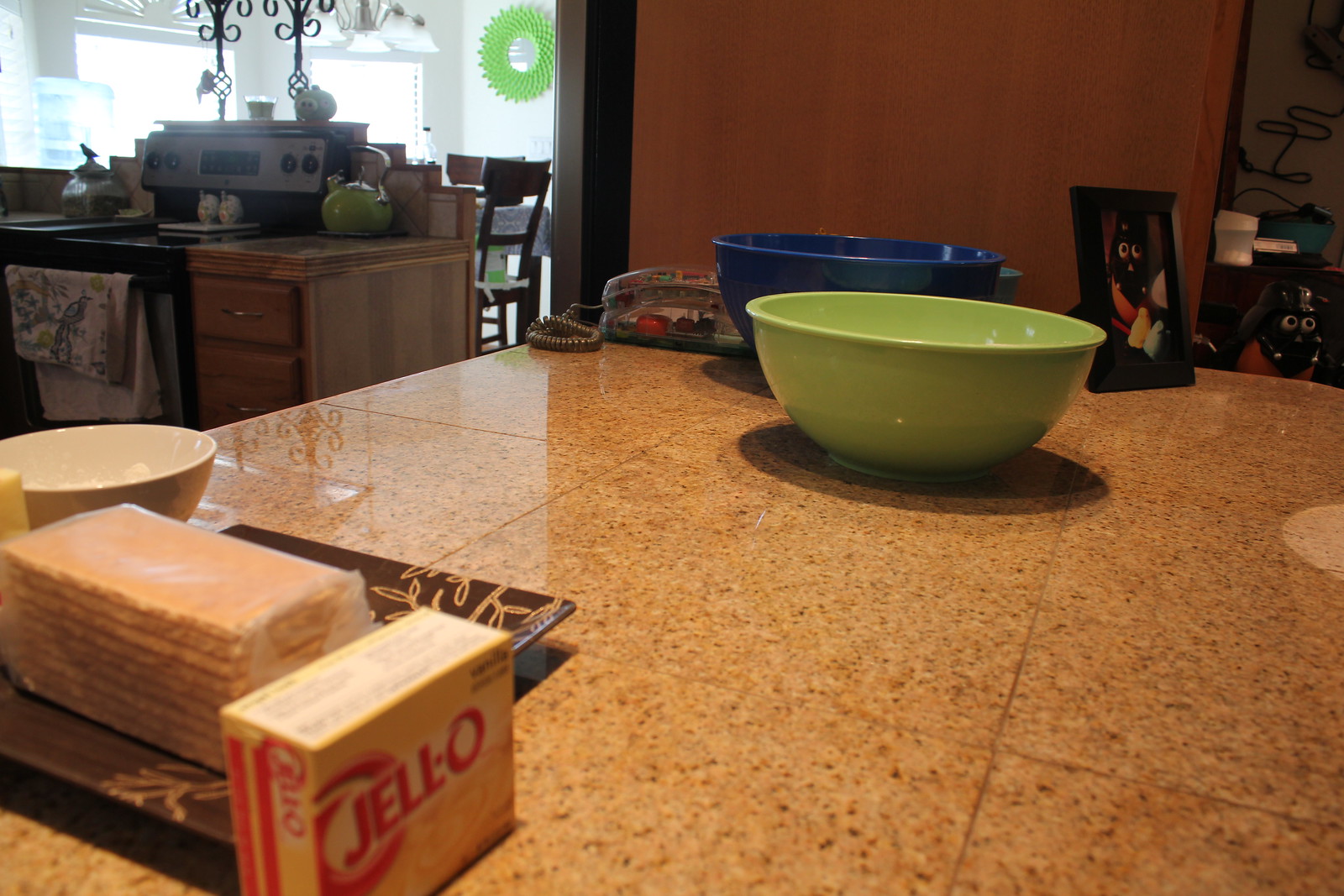In the photograph of a kitchen's marble countertop, various food items are carefully arranged. On the left side of the image's foreground, a square, flat plate is prominently displayed, bearing a package of long, rectangular crackers. In front of this plate, a small box of Jell-O in vibrant yellow and red hues partially obscures one of its corners. Centrally positioned on the countertop is a light green bowl, which is noticeably situated in front of a blue bowl. Further in the background, towards the top left corner of the image, the kitchen setup includes a black oven with a towel draped over its handle.